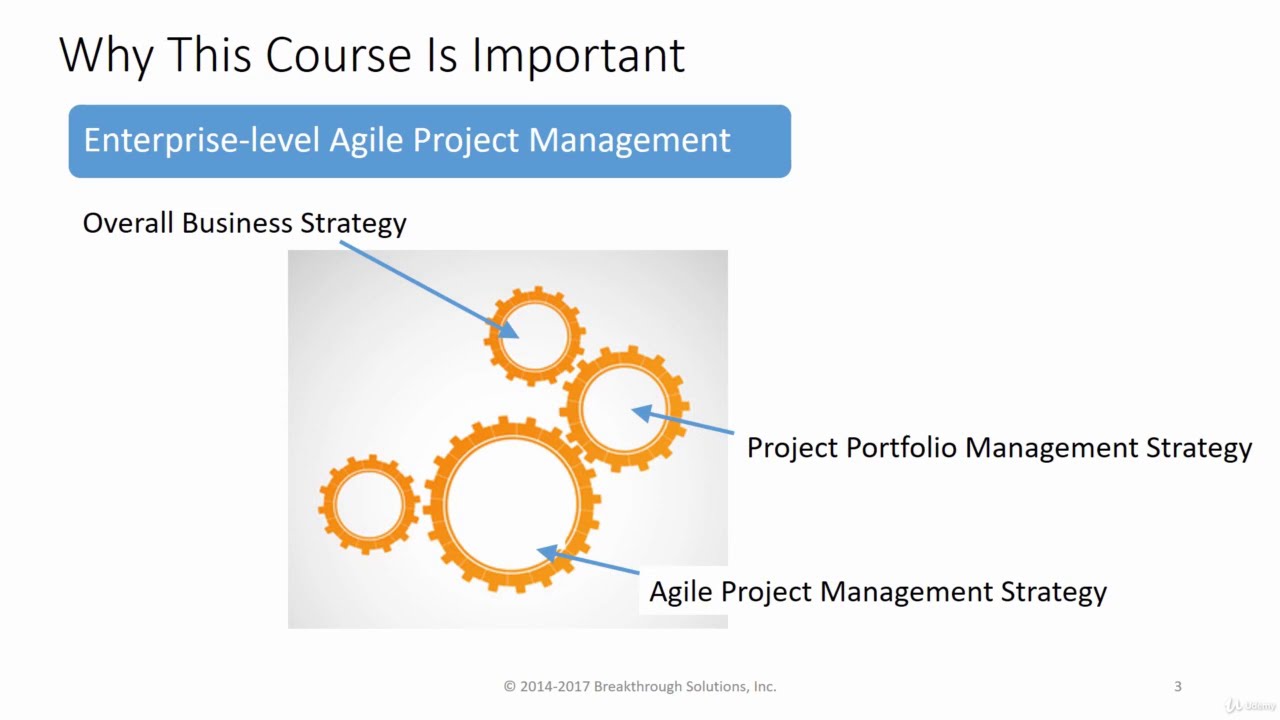The presentation slide features a clean white background and is centrally focused on a visual and textual explanation of the importance of an Enterprise-Level Agile Project Manager course. At the top, black text reads "Why This Course Is Important." Below this, a light blue box with white letters highlights "Enterprise Level Agile Project Manager." In the center is an image of interconnected gears in gray and orange hues, each representing a different strategic element. The first small gear, with an arrow pointing to it, is labeled "Overall Business Strategy" in black letters. The second gear, connected by another arrow, is termed "Project Portfolio Management Strategy." The largest gear, highlighted with a blue arrow, represents the "Agile Project Management Strategy." The color scheme consists of gray, black, white, blue, and orange, and together, the elements convey how various strategies interlink to illustrate the course’s significance, akin to an educational textbook or presentation slide.